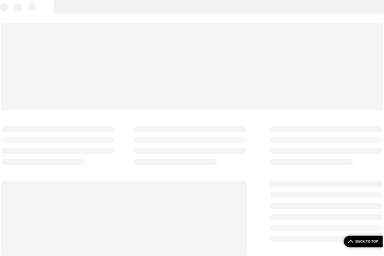This is a grayscale mock-up of a web page set against a white background. Dominating the bottom right corner is a small black rectangle featuring the text "back to top" in white. The mock-up lacks any written content, save for the "back to top" text. The page is sectioned off to indicate areas meant for future text and photos. At the very top, there's a space resembling a browser address bar. Aside from these structural placeholders, the image is devoid of any actual photos, illustrations, people, plants, animals, or buildings. The image overall is minimalist, focusing purely on the layout without any decorative elements or distractions.